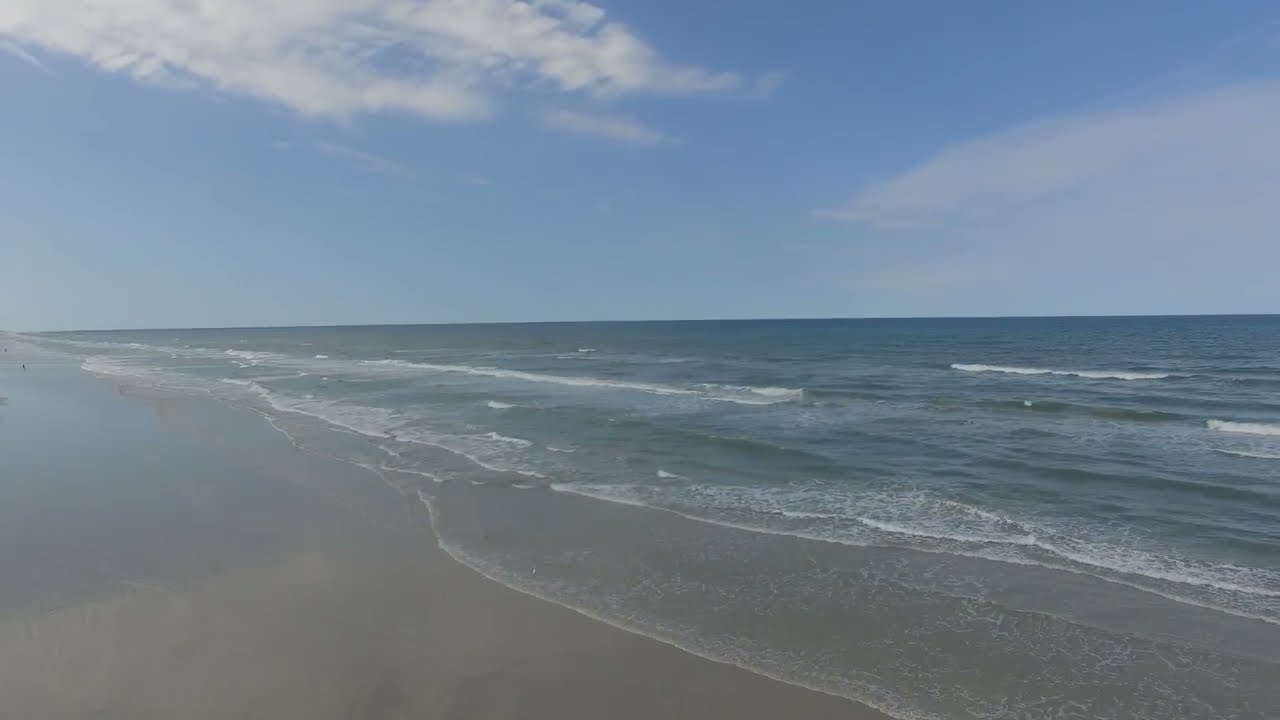The image depicts a vast seascape with a serene beach located on the left-hand side. The ocean stretches out endlessly to the horizon with no land in sight. Gentle waves, no more than a foot tall, softly lap against the grayish-tan sandy shore, which, while wet from the waves, appears devoid of any visible shells or stones. The sky overhead is a clear blue with a few wispy high clouds, giving the impression of a bright yet slightly hazy day. A single fluffy cloud is noticeable at the top left of the image. There are no boats, lighthouses, or visible marine life present, emphasizing the tranquil and undisturbed nature of the scene. Though the beach is mostly empty, a tiny, indistinct figure can be seen far off in the distance on the left. Overall, the image captures a peaceful, expansive oceanfront setting under a partly cloudy sky.